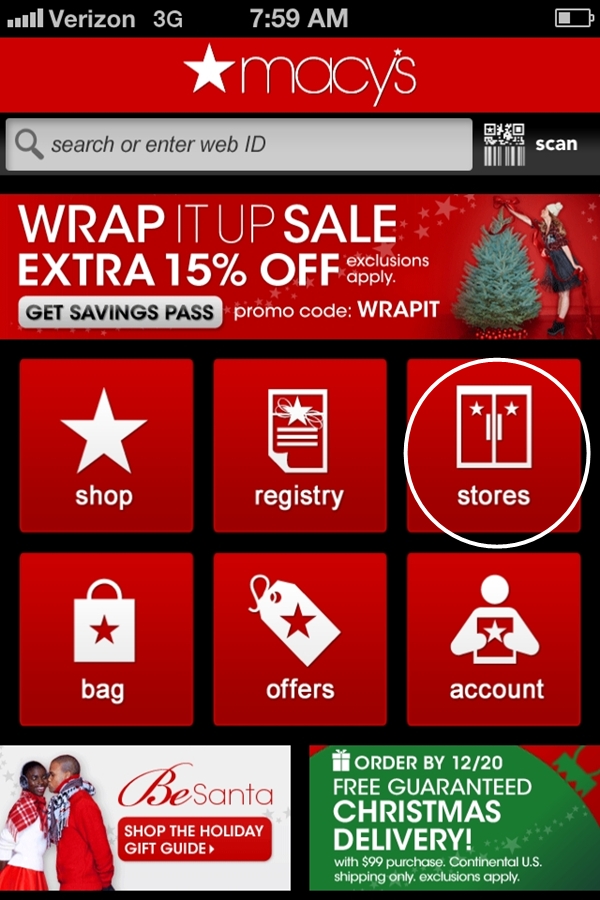A smartphone screenshot showcases the Macy’s website, prominently displaying various details and features. The device's status bar shows it's 7:59 a.m., with icons for battery, signal strength, and a 3G network provided by Verizon. The website's header has a red background with the Macy’s logo, a white star, and a search box labeled "search or enter web ID." To the right of the search box is a QR code with a "scan" button.

Below the search bar, a red advertisement banner announces a "Wrap it up sale" offering an extra 15% off, with specific exclusions. The banner also includes a promo code "WRAPIT" and an image of a girl decorating a Christmas tree, further enhancing the festive theme.

Centered beneath the advertisement, six red and black icons represent various categories: 

1. "Shop" with a white star.
2. "Registry" with a white clipboard.
3. "Stores" with two white windows, encircled by a white ring.
4. "Account" showing a person holding an object.
5. "Offers."
6. "Bag" depicted with a bag icon.

At the bottom, two additional ads appear. The left ad features a Santa theme, urging users to "Be Santa" and explore the holiday gift guide. The right ad, green in color, promises guaranteed Christmas delivery for orders placed by December 23rd with a $99 purchase, applicable to continental US shipping only and subject to exclusions.